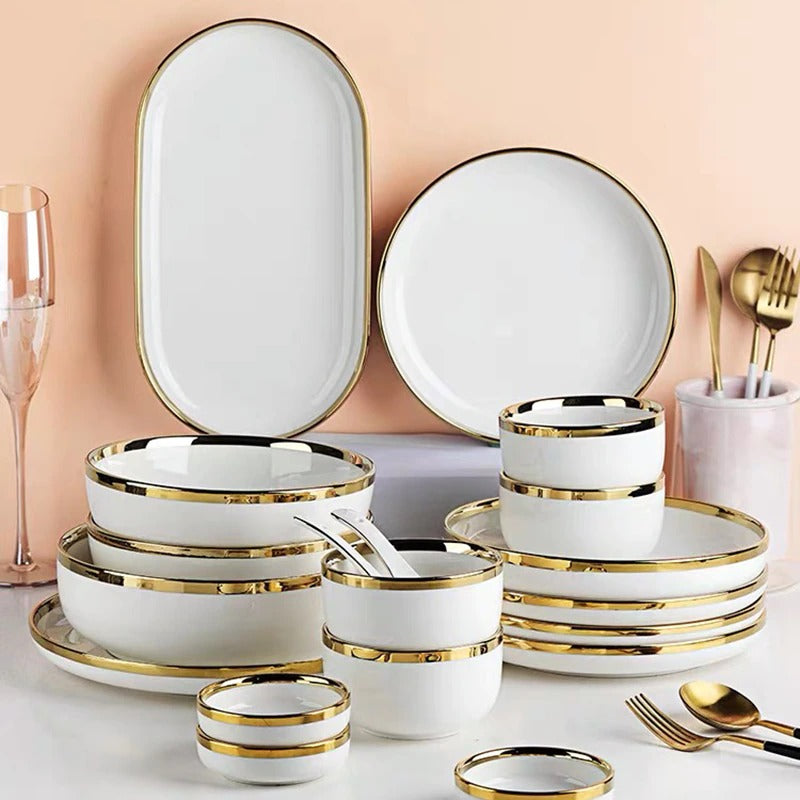This close-up image showcases an artful arrangement of elegant, matching dishware on a pristine white tabletop set against a soft peach-colored wall. The dish set, predominantly white with a delicate gold trim, includes various plates, bowls, serving dishes, and a champagne glass filled with ice on the far left. On the right side, there's a neat stack consisting of four plates with two bowls perched atop. The left side features another plate supporting a few nested serving bowls and smaller sauce bowls. Centrally, there are additional bowls with white-handled serving utensils peeking out. Along the bottom right, sophisticated golden silverware with black detailing at the midsection is laid out. Leaning against the wall in the upper part of the image, there's a large oval platter and a white plate arranged upright, accompanied by a white holder containing a gold knife, spoon, and fork. This carefully composed scene highlights the set's cohesive design and chic aesthetic.